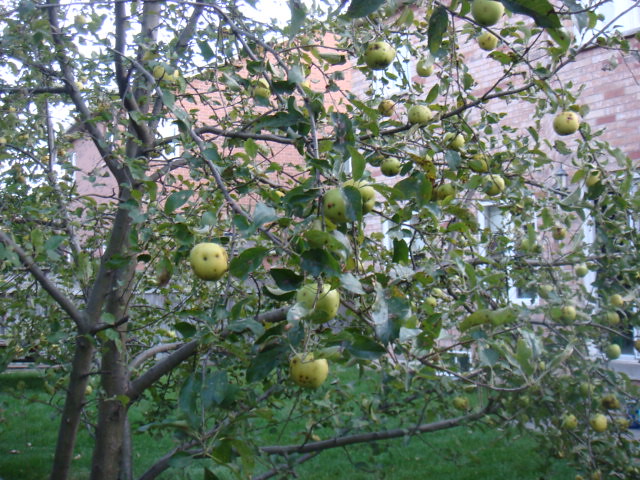In the foreground of this detailed photograph, a sparsely-leaved, thin-branched apple tree stands laden with small, light green apples, many of which show signs of bruising and nibbling from worms and other critters. The apples, scattered mostly on the right side of the tree, present a lime yellowish-green hue. Beneath the tree, lush green grass sprawls across the base. Behind this main feature, a brick facade house with white trim dominates the background, flanked by a similar neighboring red brick house with white trim, both buildings partially obscured by the tree canopy. A daylight sky washes over the scene, casting a soft light that highlights the contrasting textures and colors, while a privacy fence demarcates the boundary between the two yards.